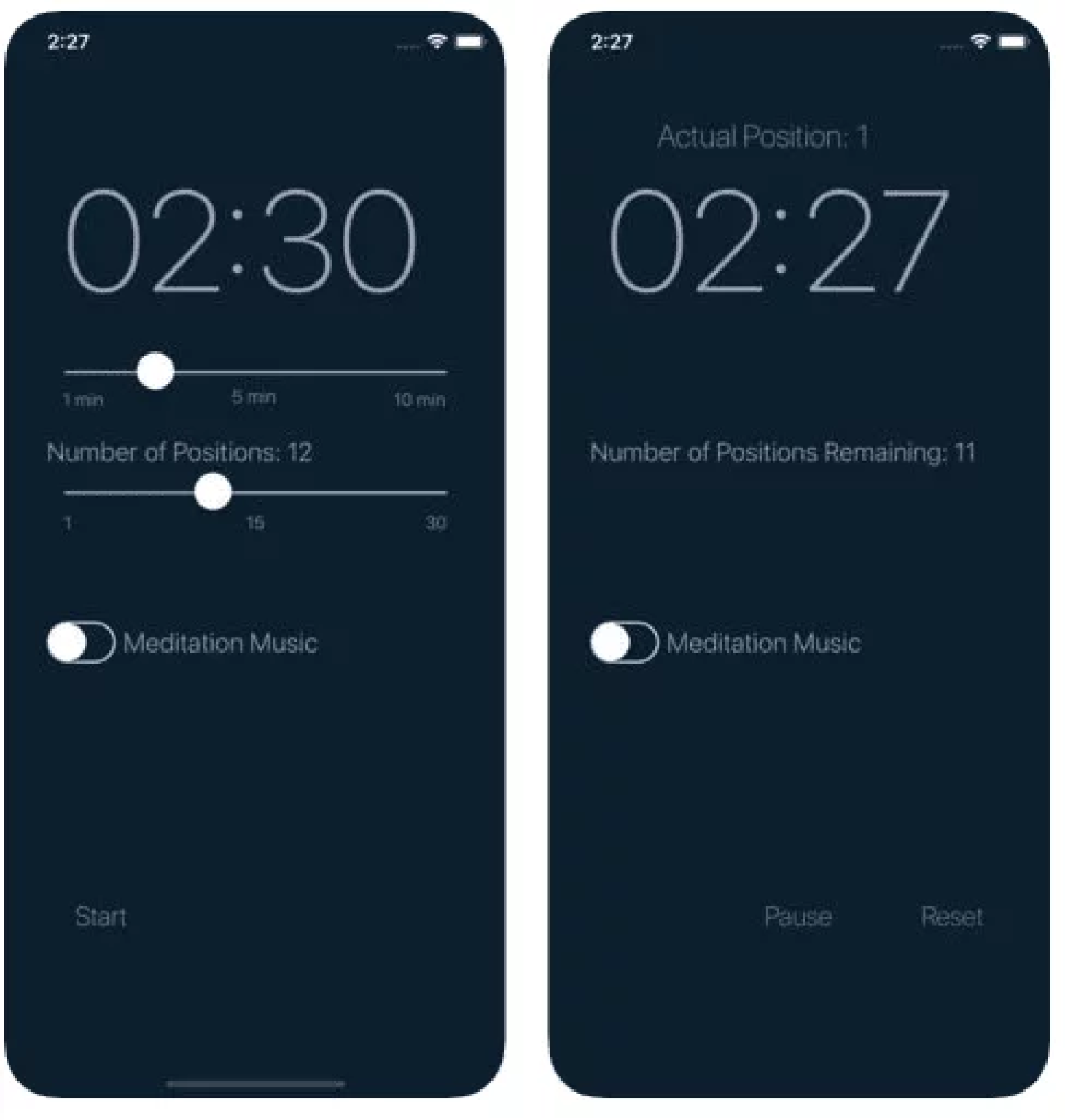The image displays two smartphone screens side-by-side, both featuring a dark background in a shade close to midnight blue. Each screen shows 2:27 AM at the top left, with Wi-Fi and battery icons on the top right.

The left screen prominently displays "02:30" in large numbers, indicating 2 minutes and 30 seconds. Below the time, there is a slider bar marked for duration settings: 1 minute, 5 minutes, and 10 minutes, with the slider set around the 2 to 3-minute mark. Another slider beneath is labeled "Number of positions 12" and ranges from 1 to 30, with 12 being highlighted. Below these, there is a toggle switch for "Meditation music," which is turned off. Toward the bottom of the screen, a "Start" button is visible.

The right screen shows "02:27" in large numbers, indicating 2 minutes and 27 seconds, with the text "Actual position 1" above the time. The phrase "Number of positions remaining 11" is displayed, suggesting a sequence in progress. Meditation music remains toggled off. Instead of a start button, it features "Pause" and "Reset" buttons, indicating an active session.

Both screens appear to be part of a wellness or yoga app, providing time-based session controls and monitoring the number of positions in the routine.